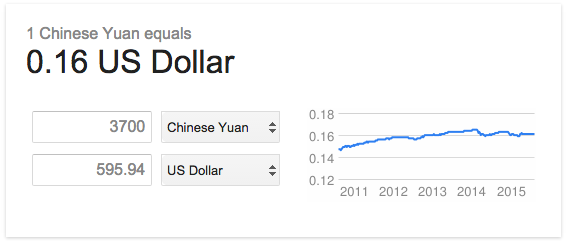The image features a white rectangle with a gray outline. In the top left corner, "1 Chinese YUAN = 0.16 US dollar" is prominently displayed, with "0.16 US dollar" in bold black text beneath "Chinese YUAN" in gray.

Below this, on the left side, are four smaller rectangles: the first two have gray outlines and white backgrounds with black text stating "3,700" and "595.94" respectively. The next two rectangles are filled gray with black text, labeled "Chinese YUAN" and "US dollar." On the right side of these gray rectangles are up and down arrows.

To the right of these elements is a chart depicting the exchange rate trend of the US dollar to the Chinese Yuan from 2011 to 2015. The vertical axis starts at 0.18 and descends to 0.12 in 0.02 increments, while the horizontal axis marks the years 2011 through 2015. Gray horizontal lines correspond to each 0.02 increment on the vertical axis. A blue, squiggly line illustrates the fluctuating exchange rate, rising and falling between 0.14 and 0.18 over the five-year period.